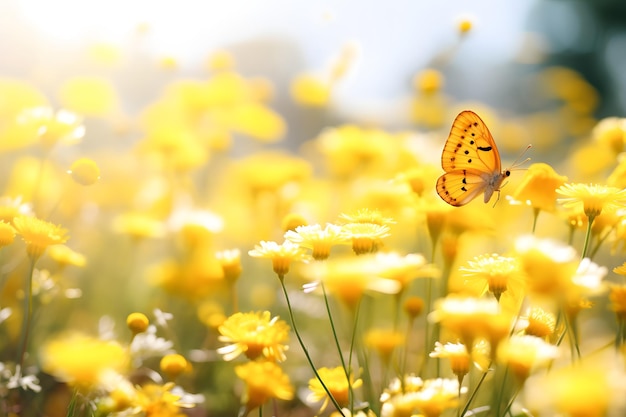This close-up image captures an enchanting field of yellow flowers under bright, sunny skies, bathed in a glossy sheen suggestive of early morning dew. The background is a blur of bright yellow flowers, creating a bokeh effect that fades into indistinct shapes, adding to the dreamy quality of the scene. The focal point of the photograph is sharply on the right side, where a stunning butterfly alights on one of the flowers. The butterfly, primarily yellow with intricate orange and black patterns on its wings, has orange dots outlining the edges and a series of black lines and dots near the top. Its yellow body is adorned with delicate black accents, and its antennae elegantly extend forward. This detailed composition, whether a skillful photograph or AI-generated masterpiece, draws the eye immediately to the vivid butterfly amidst the expansive field of blurred yellow blossoms.